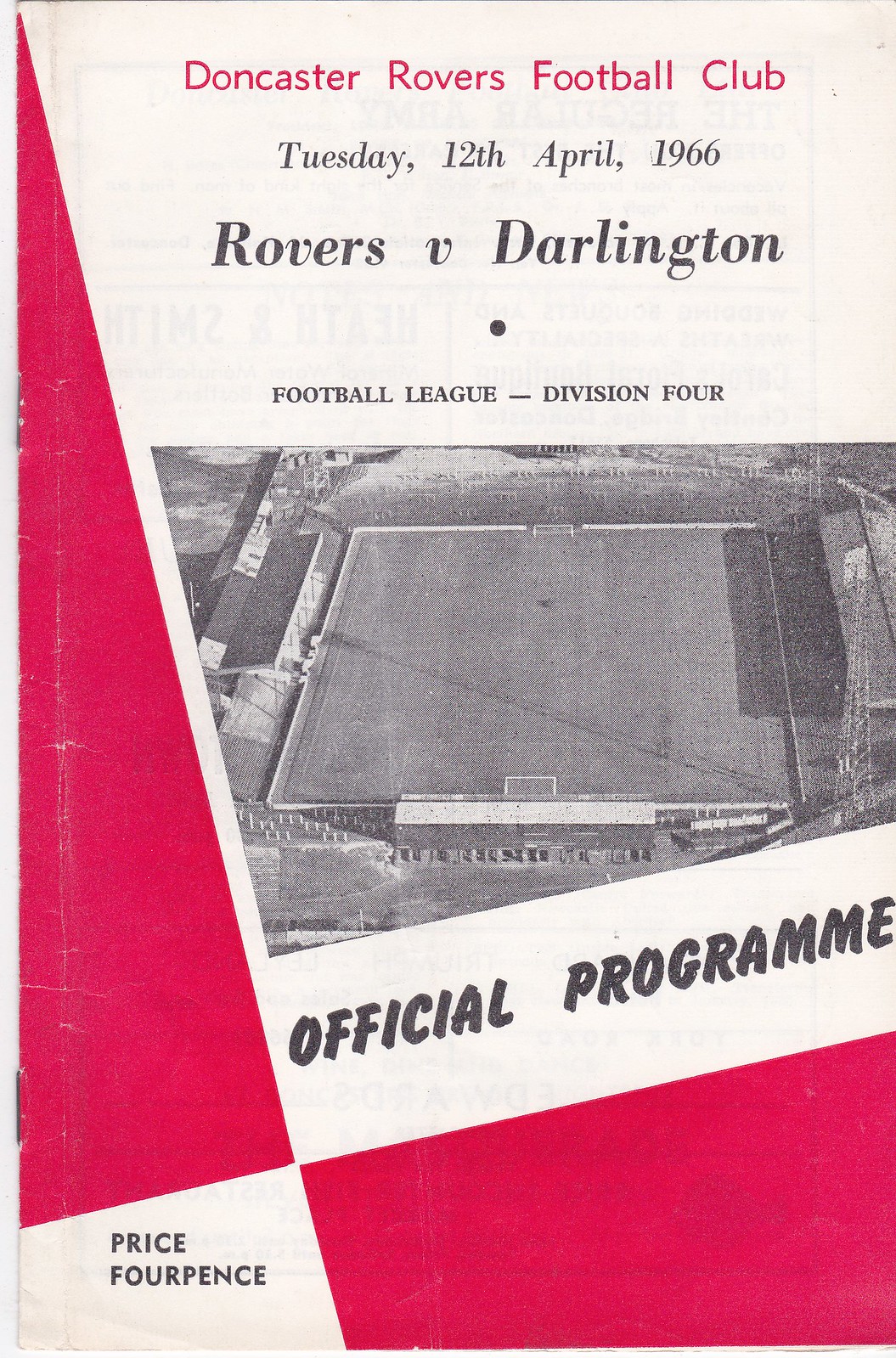This is the cover of an official program for a soccer match featuring the Doncaster Rovers Football Club. At the top of the cover, on a faded pinkish-white background, "Doncaster Rovers Football Club" is written in striking red. Below that, in black text, the date "Tuesday, April 12, 1966" is displayed, followed by "Rovers vs. Darlington" and "Football League, Division IV." Central to the cover is a large, black-and-white photograph showcasing an overview of the stadium, mainly highlighting the pitch with visible goals at either end and some of the stands. Beneath the photo, a white-striped section features the text "Official Program" in black. The bottom left corner of the cover contains a small white square with the text "Price 4 Pence" in black. The cover also includes decorative red triangles and shapes along the bottom right and left edges. The program appears to be worn and stapled together.